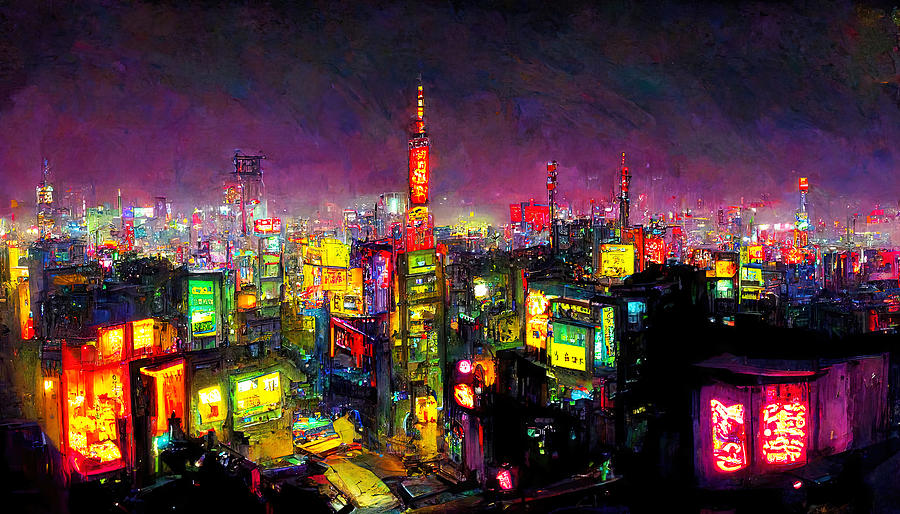This painting depicts a vibrant cityscape at night viewed from an elevated perspective, possibly from another skyscraper. The upper 40% of the image is dominated by a gradient night sky that transitions from deep black at the top to a glowing mix of pink, purple, and midnight blue as it nears the horizon. Below, an array of skyscrapers and buildings of varying heights and shapes fill the scene, painted in a representational style using a palette of neon colors—primarily purples, pinks, yellows, greens, and reds. The brightly lit building façades and streetlights cast a vivid glow that contrasts with the darker edges framing the scene, suggesting a city brimming with life despite the absence of visible people or vehicles. The buildings feature illuminated windows, red towers, and colorful signage, exuding an electric urban energy. A curved, illuminated wall in the right foreground adds to the composition's dynamic visual interest. While not photorealistic, the visible brushstrokes and geometric forms give the painting a lively, abstract quality, possibly rendered in oil.